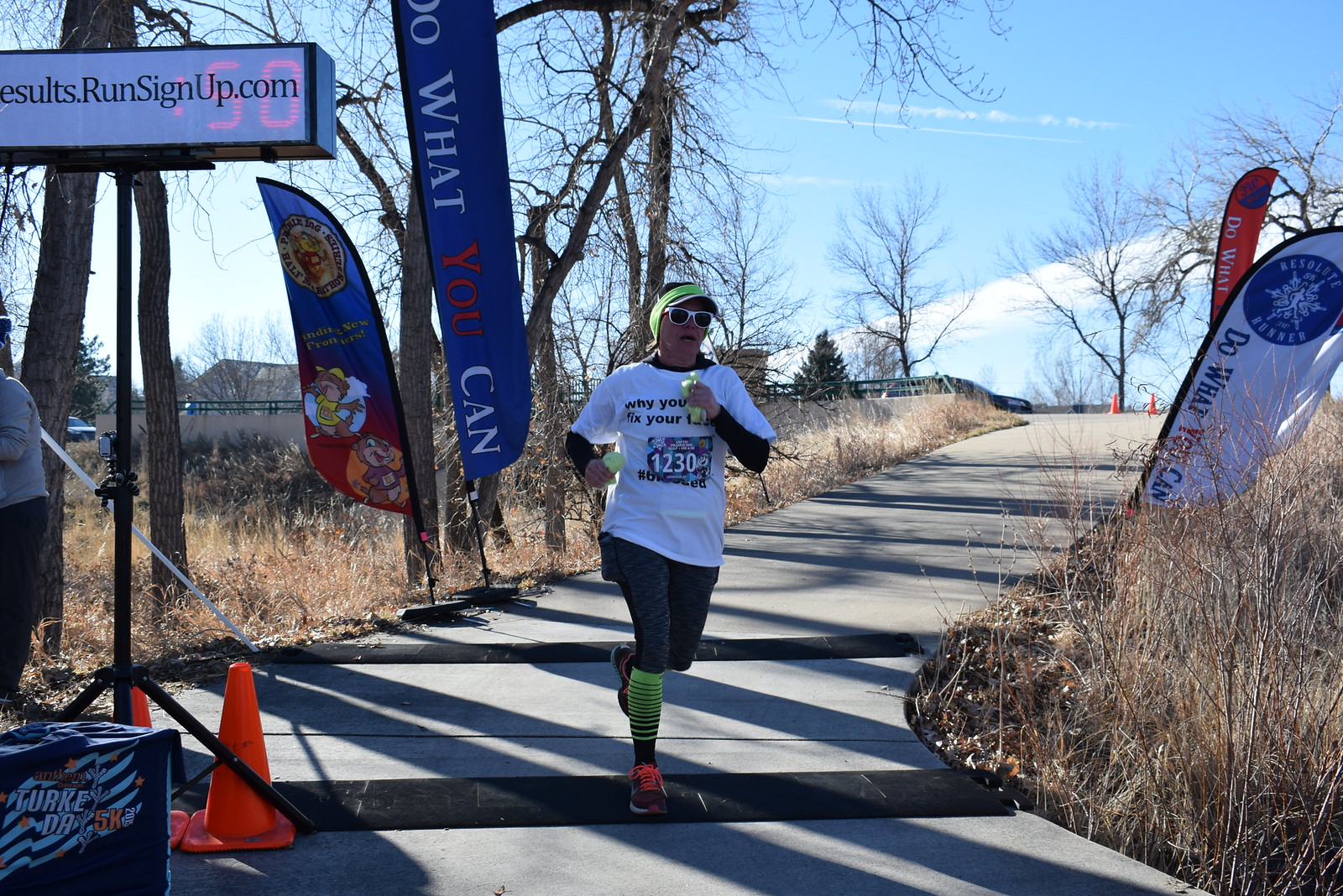The photograph captures a woman running along a concrete path during what appears to be a marathon or a sprint event held outdoors on a sunny day with a few clouds in the sky. The woman is wearing a white short-sleeve t-shirt with the number "1230" pinned to it over a black long-sleeve undershirt. She also sports white sunglasses, a black and white cap with a green headband, and black leggings. Her footwear includes black tennis shoes with orange laces, complemented by long black and fluorescent green striped socks. Surrounding her on both sides of the path are various banners and flags in blue, white, and other colors, some of which display motivational phrases like "do what you can" in different colored text (blue, white, and red).

On the left bottom corner, a couple of orange caution cones are visible, and a digital sign reads "results.runsignup.com," indicating the official timing system. The background features overgrown fields of dried-up grass, a distant building, and several trees, suggesting that the event takes place during winter. Overall, the image captures the energetic atmosphere of a running event set against a backdrop of natural and man-made elements.